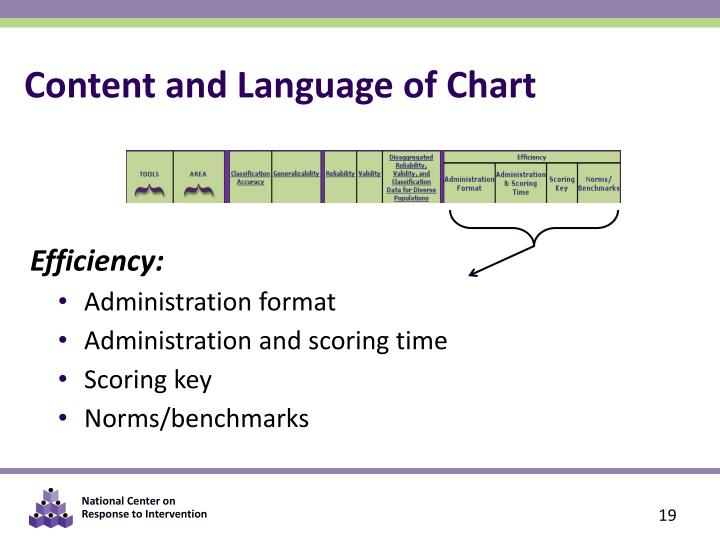The image is of a multi-color print piece prominently titled "Content and Language of Chart" at the top in bold letters. Just below, slightly off-center to the right, there is a horizontal green rectangle with blue printing, densely packed with small text. The text includes various categories and terms such as tools, areas, classification, accuracy, generalization, reliability, validity, administration format, scoring key, and data for diverse populations. Below this section, the word "efficiency:" is printed in black, followed by four bullet points: Administration format, administration and scoring time, scoring key, and norms/benchmarks. At the bottom of the chart, a small purple logo reads "National Center on Response to Intervention," with the number 19 located in the bottom right corner.